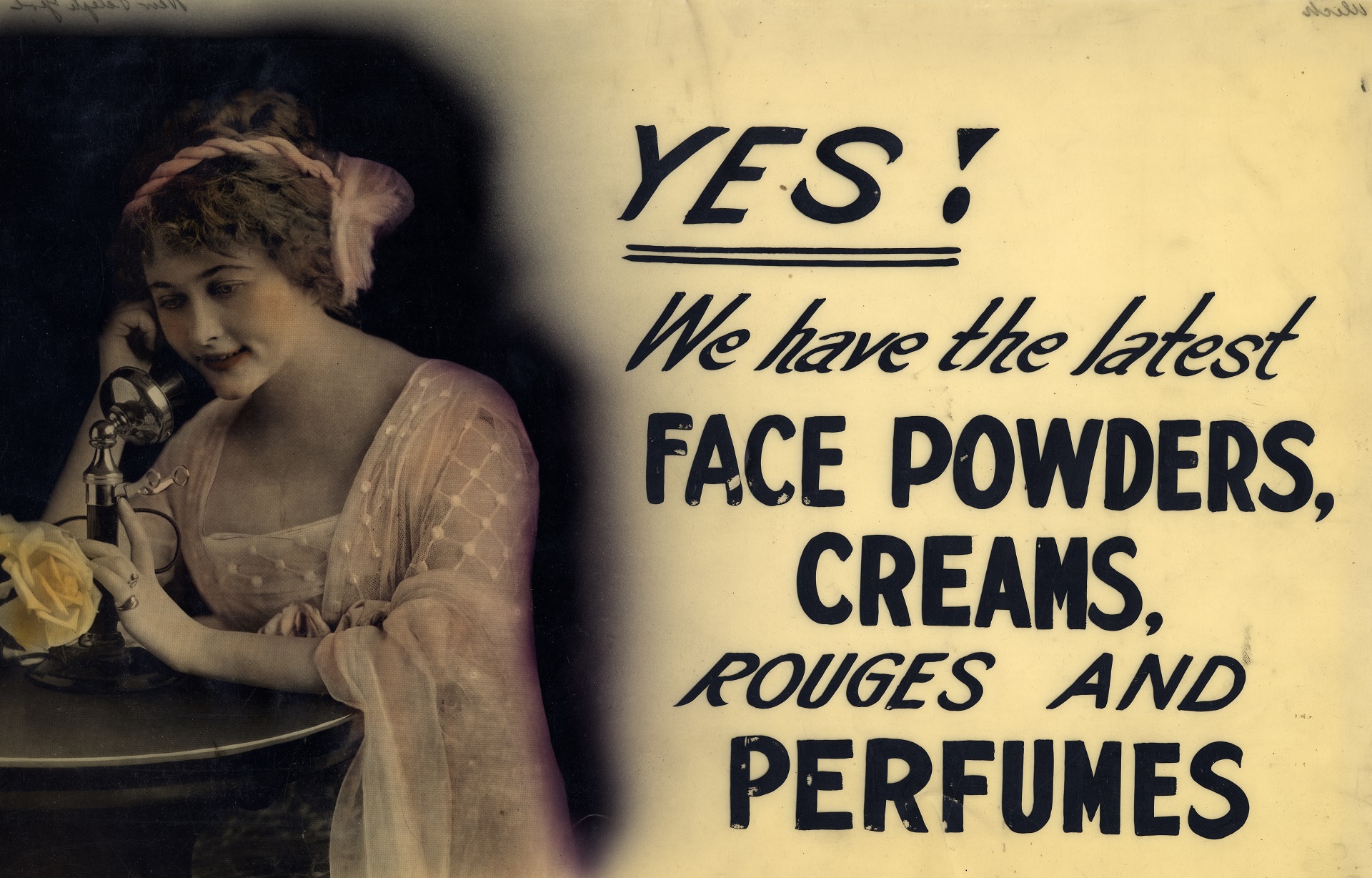The image is an old-style advertisement poster from the early 20th century, featuring a realistic drawing of a young woman standing and talking on a vintage phone on the left side. The woman is dressed in cream-colored, sheer clothes and a headband, with a yellow rose and a round table with the old-fashioned telephone in front of her. She has subtly colored rosy cheeks, adding to the nostalgic aesthetic. The background of the woman is black, which contrasts with the right side of the poster where a sepia-toned area showcases dramatic, black text. The prominent, underlined word "Yes!" heads the text, followed by a statement in bold font: "We have the latest face powders, creams, rouges, and perfumes."